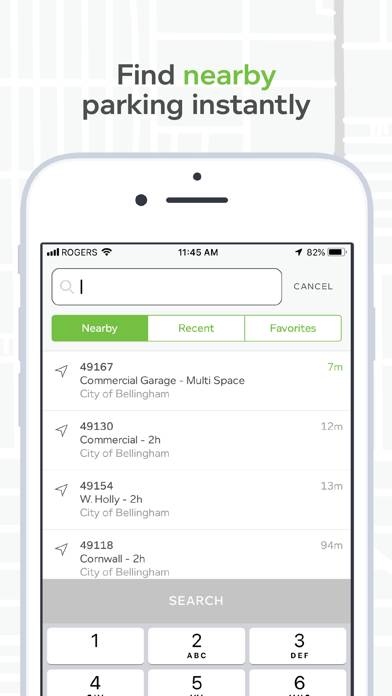A detailed description of the image:

The image features an iPhone displaying an application that appears to be a navigation or location-based app for finding nearby places. The app interface has a minimalist design with a predominantly white and light gray background accented by light green elements. At the top of the screen, there is a search bar with a flashing cursor, indicating that the user is about to enter a query. Though no text has been typed yet, the application is already showing an array of initial search results below the bar, all of which are commercial buildings identified by numbers, but not particularly useful without more context.

The screen also displays a virtual keyboard at the bottom, ready for input. The keyboard layout includes visible numeric keys: 1, 2, 3, 4, 5, and 6. The app interface suggests that search results dynamically update as the user begins typing, likely refining the list to display more relevant locations such as stores or landmarks based on the input text. For instance, typing 'WAL' might bring up results such as Walmart. The overall clean and user-friendly design implies ease of use for locating various places.